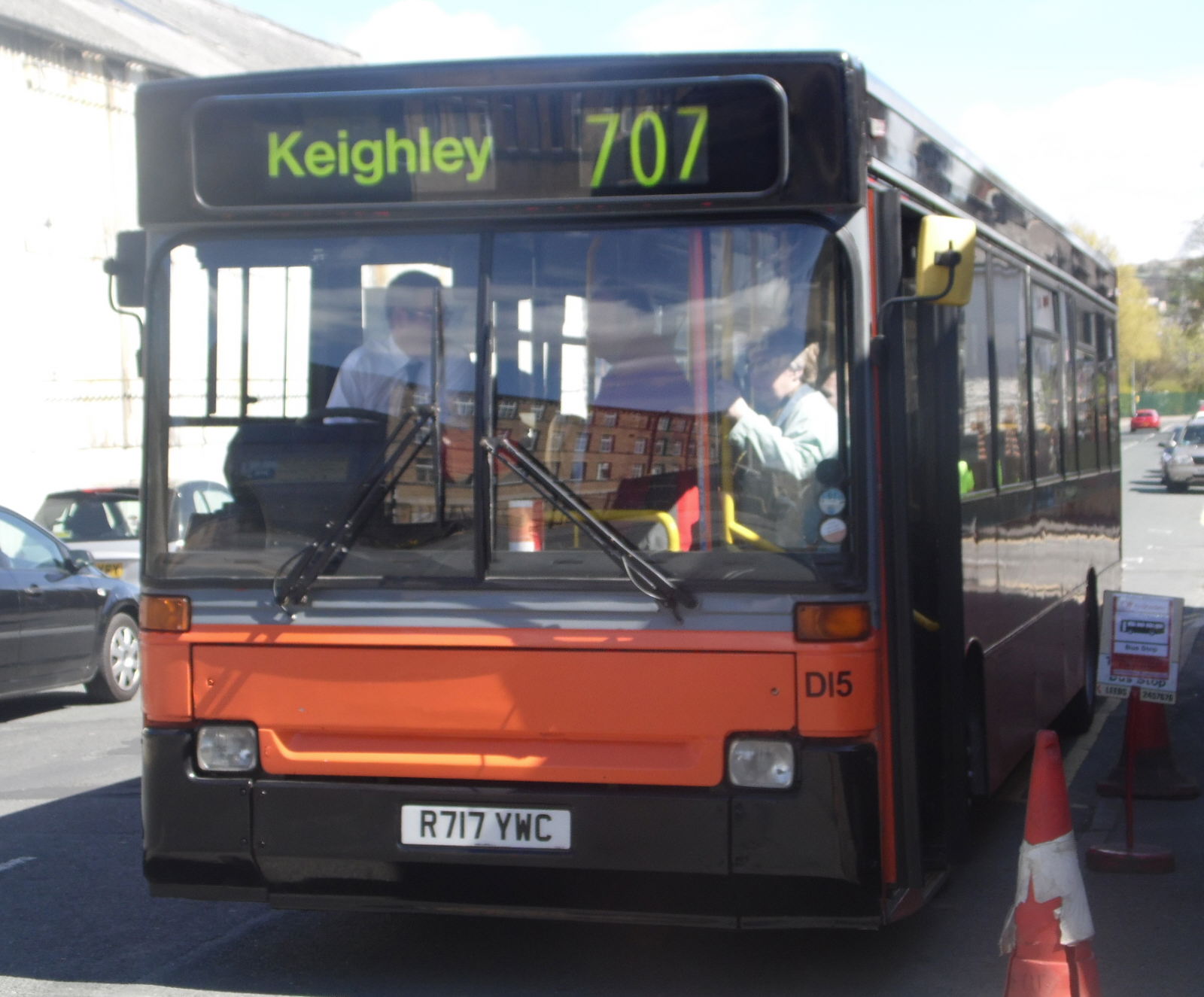The photograph, taken outdoors during the daytime, captures the front end of a parked black bus, slightly wider than it is tall. On the bus's front display in green print, it reads "Keighley 707." The bus features large front windows, with the driver visible behind the windshield, seemingly engaged in conversation with a passenger. Below the windshield, the bus is painted a reddish-orange, transitioning to black underneath the lights. The white license plate displays "R717YWC." In the right-hand corner, against a red background and beneath an orange light, the number "D15" is visible.

To the right of the bus, yellow and orange construction cones are placed on the ground. The background reveals a street with parked cars, a part of a building on the left, and fragments of a black and a white car. Above, the image is framed by a bright blue sky with scattered white clouds, adding a touch of serenity to the bustling street scene.